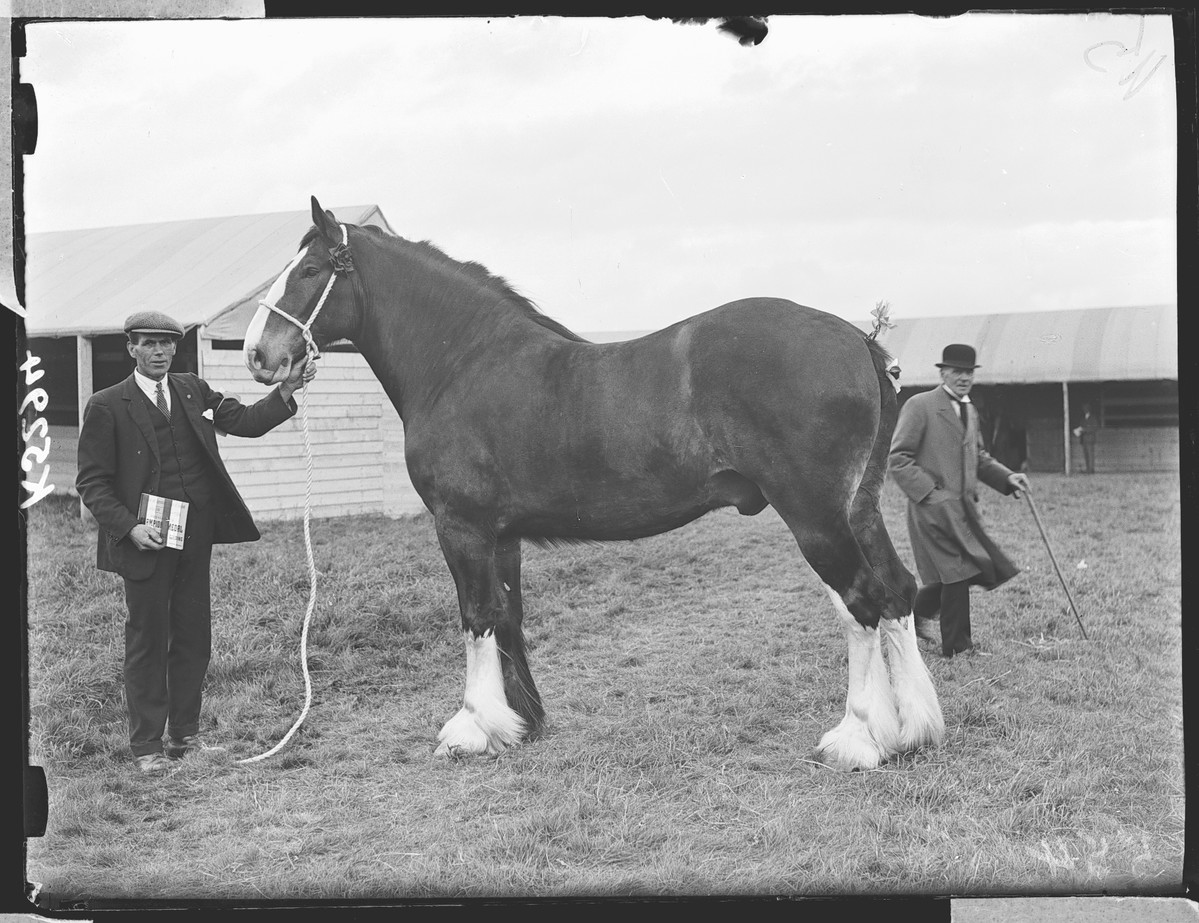In this high-quality, black-and-white photograph, measuring approximately 8 inches wide by 7 inches tall, two elegantly dressed gentlemen pose with a majestic horse outside a series of horse stables and outbuildings. The central figure, a light-skinned man in a dark three-piece suit, white shirt, and tie, with a kerchief peeking from his pocket, holds the horse with a white rope. He sports a 1920s style cap with a small brim and presents a book or pack to the camera. The horse resembles a Clydesdale or Morgan breed, with striking white lower legs, a sable body, and a distinctive white stripe down its nose, adorned with a rose by its left ear. To the right, a second man stands in a long grey overcoat, bowler hat, and tie, leaning on a cane with his left hand. The background reveals more stables and another man standing outside, reinforcing the scene's pastoral and historical setting. The photograph captures the gentlemen's and the horse's poise and elegance, emphasizing the grandeur and details of the setting.